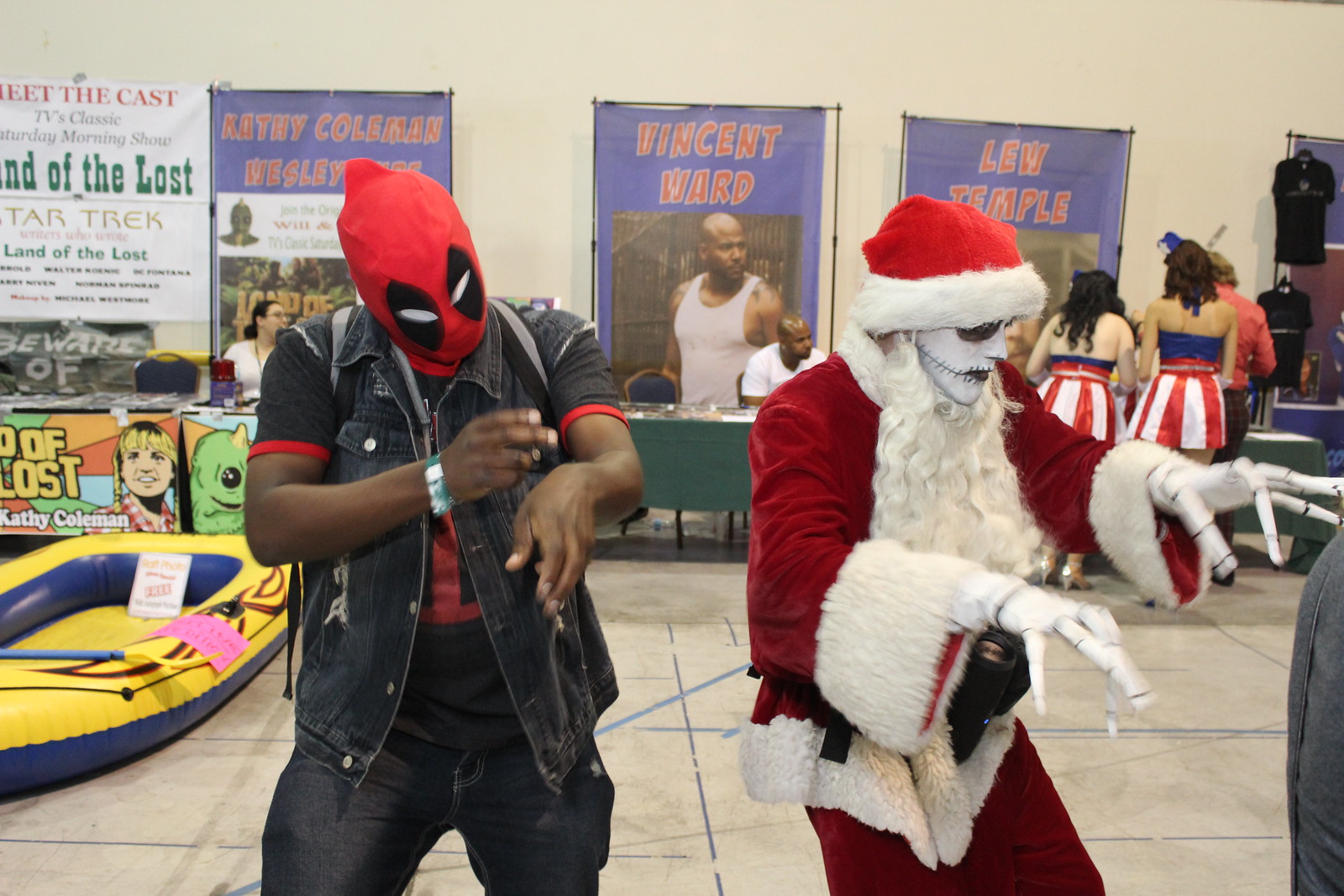In this detailed color photograph taken in a landscape orientation, the primary subjects are two men in striking costumes standing in a convention room or banquet hall. The man on the left, an African-American, is wearing a Spider-Man hat or mask that completely covers his face, a black denim vest, an orange or black shirt underneath, and blue jeans, with his arms crossed in front of his chest. His companion to the right is dressed as Jack Skellington from "The Nightmare Before Christmas," adorned in a Santa Claus costume complete with a red and white suit, a long white beard, white gloves with black lines mimicking skeletal fingers, and a skull face painted in white.

In the background is a white wall adorned with three blue banners featuring red lettering, with the central banner displaying the name "Vincent Ward" in red letters alongside a color photograph of a bald black man wearing a white tank top. The room is populated with several tables, including a central table covered with a green tablecloth and another on the left featuring a colorful cartoon drawing. In the back-right corner, several girls are seen wearing blue tank tops and red and white striped skirts, facing away from the camera. The atmosphere conveys a lively event, filled with various attendees and decorations, all contributing to the festive and dynamic scene.